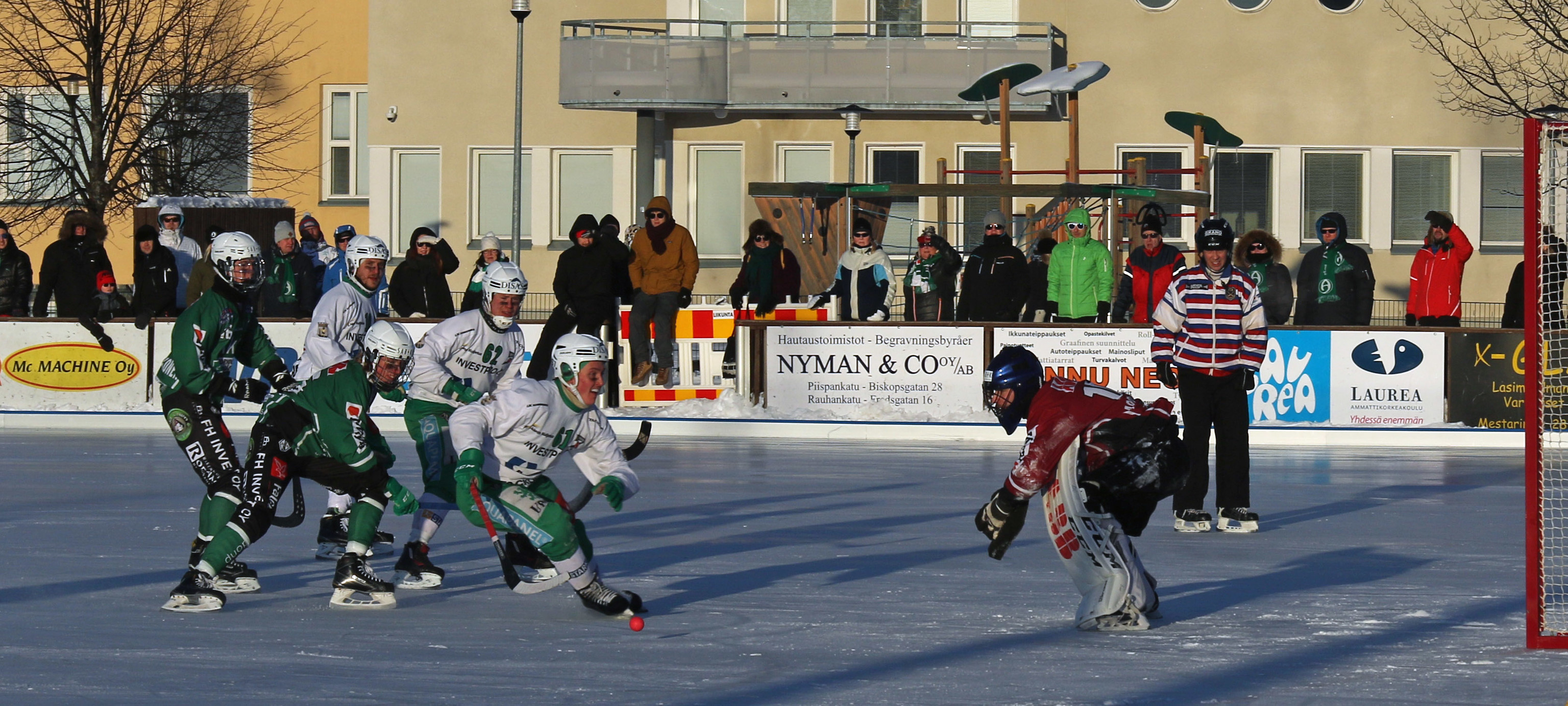The image captures an outdoor ice rink bustling with a competitive hockey game. Prominently, a group of five players, clad in a mix of white and green jerseys with white helmets and black and green pants, are intensely chasing a red puck that is mid-air, about five feet in front of the goalkeeper. The goalkeeper, wearing a red jersey and black pants with white pads, stands alert in front of the goal. Beside the goal, a referee dressed in a red and white striped shirt and black pants observes the action closely. The backdrop features several apartment buildings, streetlights, and trees, further framed by an audience of spectators standing and sitting around the rink's perimeter. The rink is surrounded by walls adorned with various advertisements such as "Niman and Company," "Loray," "Mr. Machine," and "OG," keeping the energetic scene safely enclosed.